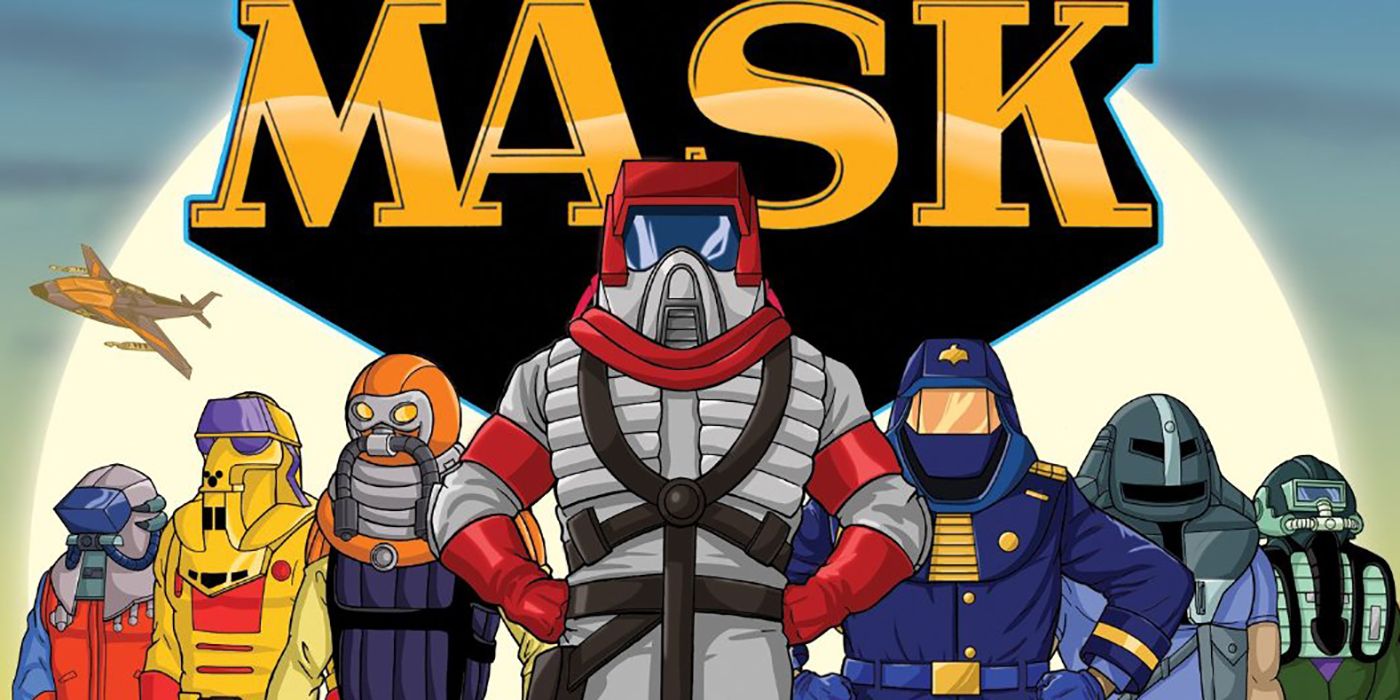This image is a detailed, drawn or computer-animated artwork resembling the title screen for a cartoon or comic. Dominating the top center, the word "MASK" is rendered in large yellow capital letters with a stylized black shadow, set against a backdrop that includes a bright white circle, akin to a moon, against a dark blue sky. To the left of the "MASK" title, a small, grey cartoon plane with yellow windows and two guns on the underside of its wings is depicted flying.

In the foreground, seven men stand in a row, each wearing various colorful and menacing space or military suits. Starting from the left, the first figure sports a blue, red, and grey suit with a blue visor. The next character is garbed in a yellow and red suit with a purple visor. The third in line dons an orange and grey ensemble with a grey chest piece. At the center stands a prominent figure in a grey suit with a red hood, red gloves, and red armbands, whose face is obscured by a helmet. To his right, another character wears a blue suit with yellow accents and a yellow visor. Moving further right, a man in a grey mask and purple shirt is depicted. The last figure on the far right wears a more rugged outfit consisting of green pants, a metal vest, and a metal helmet. All seven characters stand confidently with their hands on their hips, looking ready for action.